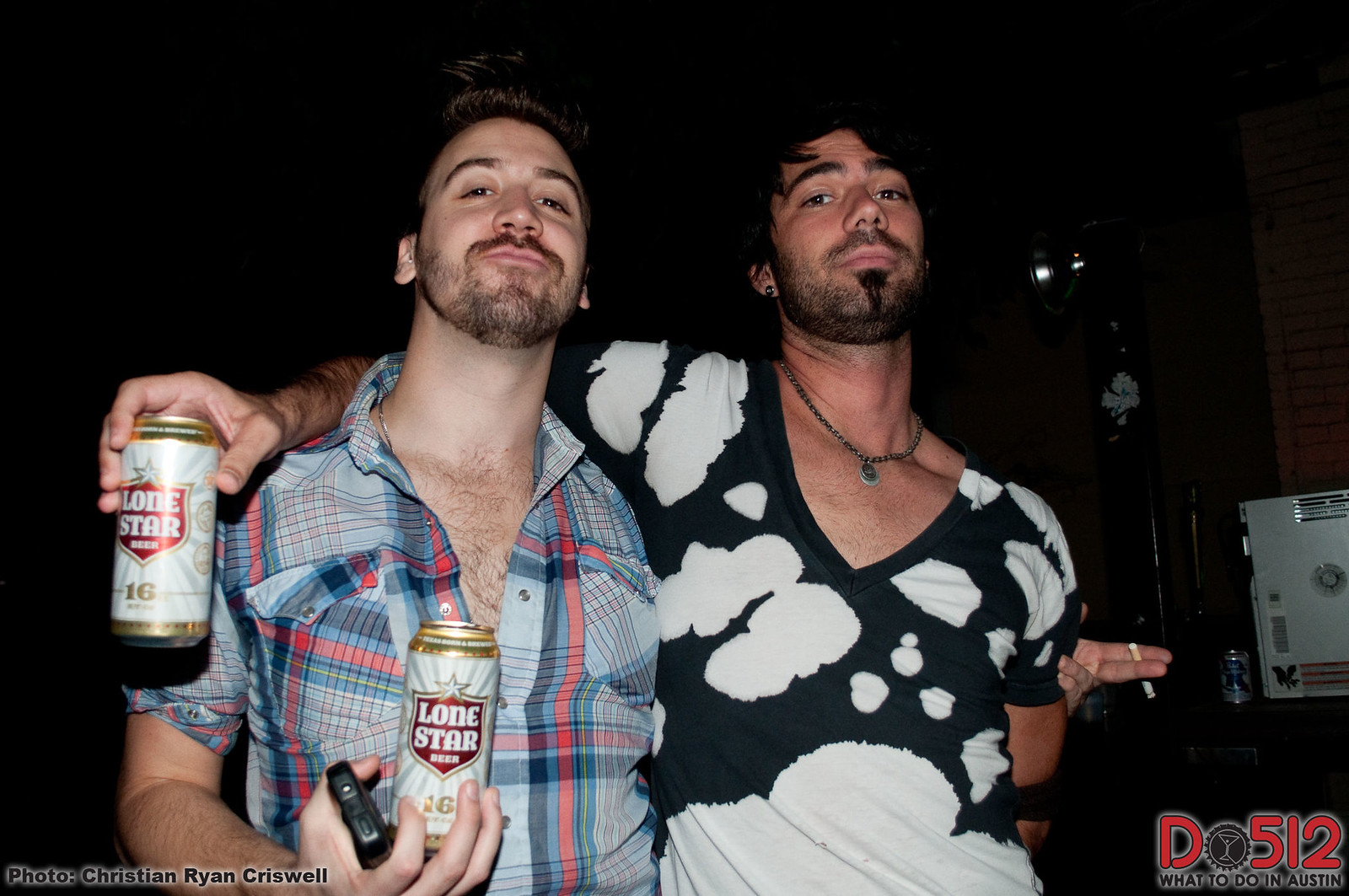In this image, two men, who appear to be twins or closely related, pose together at a dimly lit bar or club, each holding a can of Lone Star beer. The man on the left, a white male, sports a blue and red plaid button-down shirt and holds a phone along with his beer. His left hand, draped casually around the other man's shoulder, holds a cigarette. The man on the right, potentially a white or Latino male, wears a black v-neck shirt adorned with white cloud-like splotches and a silver chain necklace. He has his left arm around his friend and also holds a Lone Star beer can. The background is dark and indistinct, with a couple of lights and some metallic object, possibly a safe, bearing the logo "DO512" and what resembles an alien face. This suggests they are in an Austin, Texas, venue. The barely legible text on the lower portion of the image mentions "Criswell," though it is unclear to whom it refers. Both men gaze directly at the camera, capturing a candid moment of camaraderie.